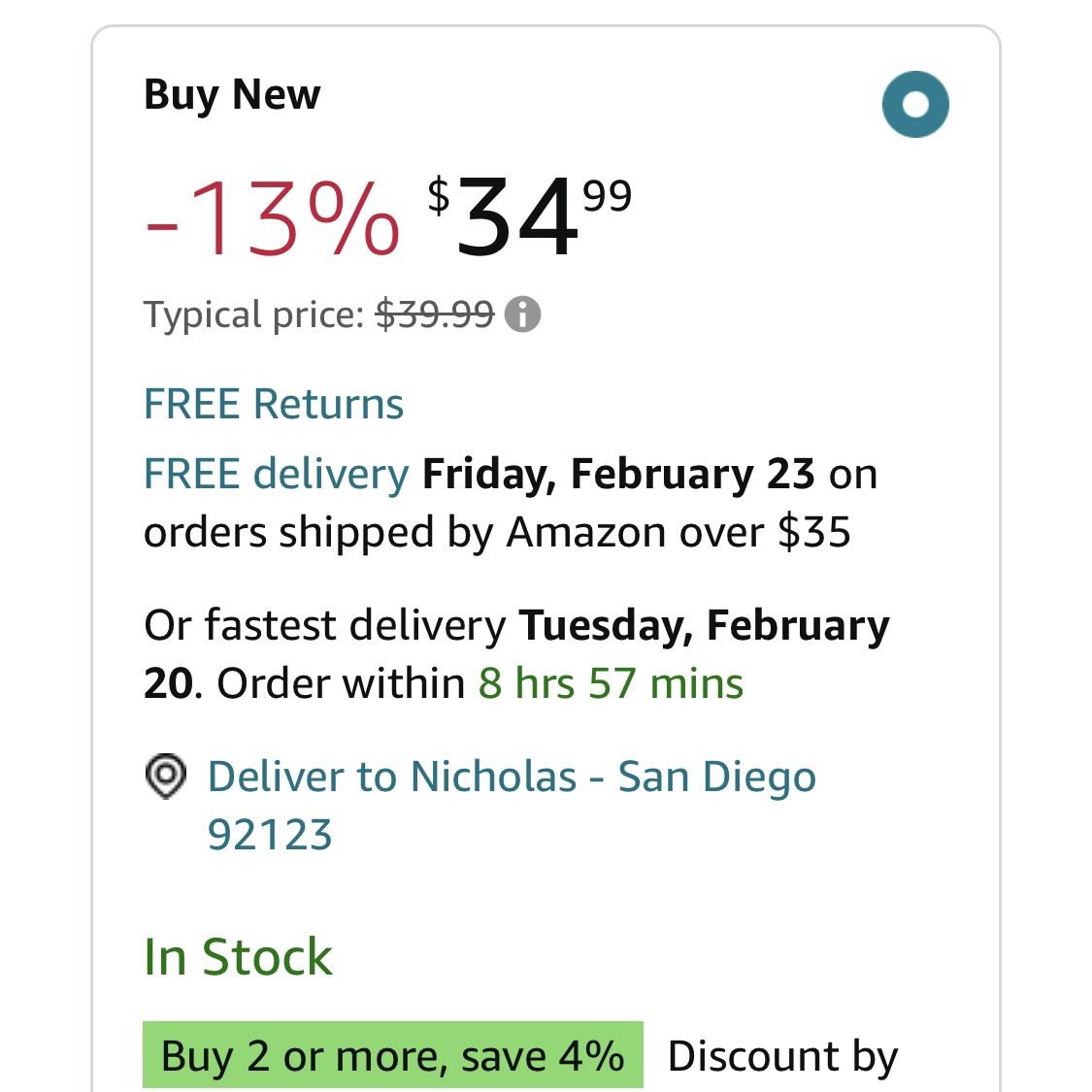The screenshot displays the price section of an Amazon product page. The current price is $34.99, reflecting a 13% discount off the regular price of $39.99, which is shown with a strikethrough next to an eye icon. The product offers free returns and free delivery, both highlighted in blue text. The expected delivery date for standard shipping is Friday, February 23rd, presented in bold black text. The item can also be delivered faster by Tuesday, February 20th if ordered within 8 hours and 47 minutes, indicated in green text. The product is available for shipping over orders of $35 and above, as mentioned in regular lowercase text. It will be delivered to Nicholas in San Diego, highlighted in blue with the accompanying map icon and zip code 9512392123. The product is in stock and sold by Tiramor, with an additional 4% saving highlighted in a green banner. The screenshot simply captures this detailed information.